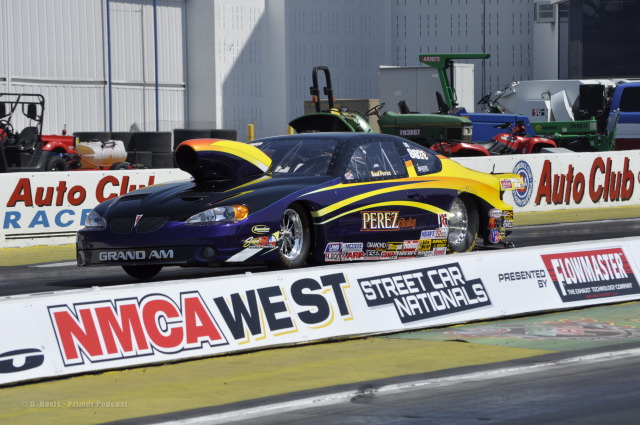This detailed photograph captures an action moment at a motorsports event, specifically the NMCA West Street Car Nationals presented by Flowmaster. The focal point is a pro-stock drag race car, a dark blue Pontiac Grand Am adorned with striking yellow racing stripes and silver chrome rims. The front of the car prominently displays the word "Grand-Am" along with the iconic Pontiac triangle emblem on the hood. 

On the side, the vehicle proudly bears the name "Perez Racing" spelled out as P-E-R-E-Z, accompanied by various smaller sponsor logos scattered along the side skirt. A distinctive feature is a large, vividly colored exhaust or engine component protruding from the middle of the hood, painted in shades of black, yellow, and orange.

In the foreground, a signboard reads "NMCA West Street Car Nationals, presented by Flowmaster," while further back another sign denounces "Auto Club Racing". The backdrop includes an array of parked service vehicles, trucks, tractors, and buildings with large garage doors, setting the scene within a bustling racetrack environment. The car, facing to the left, either has just begun its race or is preparing to do so, with both the near and distant tracks visible in the background.